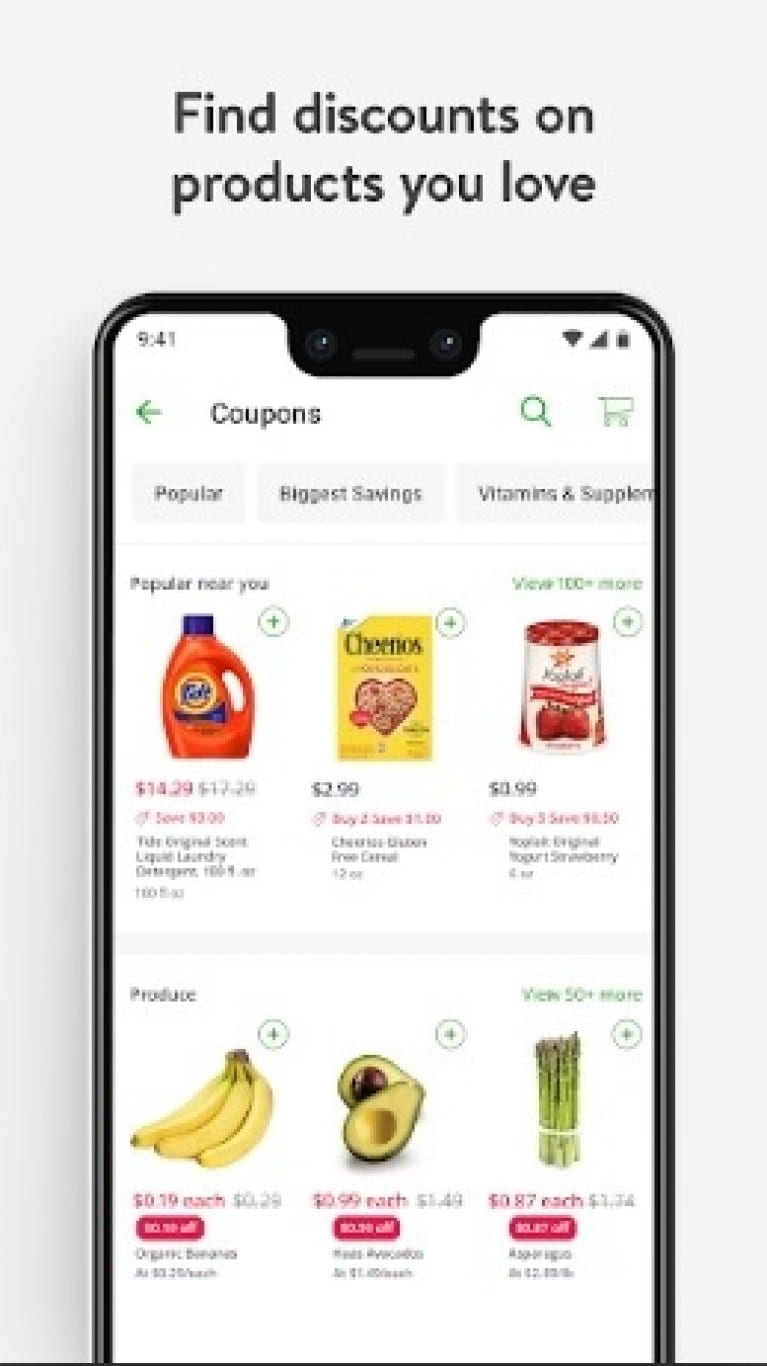This image captures a screenshot of a mobile phone displaying a coupons page, likely from the Instacart app. Positioned above the mobile phone is black text stating, "Find discounts on products you love." The mobile phone itself is sleek, featuring two front-facing cameras and a white status bar. The current time displayed is 9:41, while the top right corner shows icons for battery life, cellular signal, and Wi-Fi connectivity.

The page's header prominently displays "Coupons," and to its right are icons for a green magnifying glass and a green shopping cart. Below this header are four tags labeled: "Popular," "Biggest Savings," "Vitamins," and "Supplements."

The first section is titled "Popular Near You" and showcases three discounted items in a row:
1. Tide Laundry Detergent (Original) priced at $14.29 with a savings of $3.
2. Cheerios priced at $2.99.
3. Yoplait Strawberry Yogurt priced at $0.99.

A green link below these items invites users to "View 100+ more."

The next section highlights produce, listing:
1. Bananas for $0.79 each or $0.19 each.
2. Avocados for $0.99 each.
3. Bundles of asparagus for $0.87 each.

The entire page has a clean, white background, making the text and images easily readable.